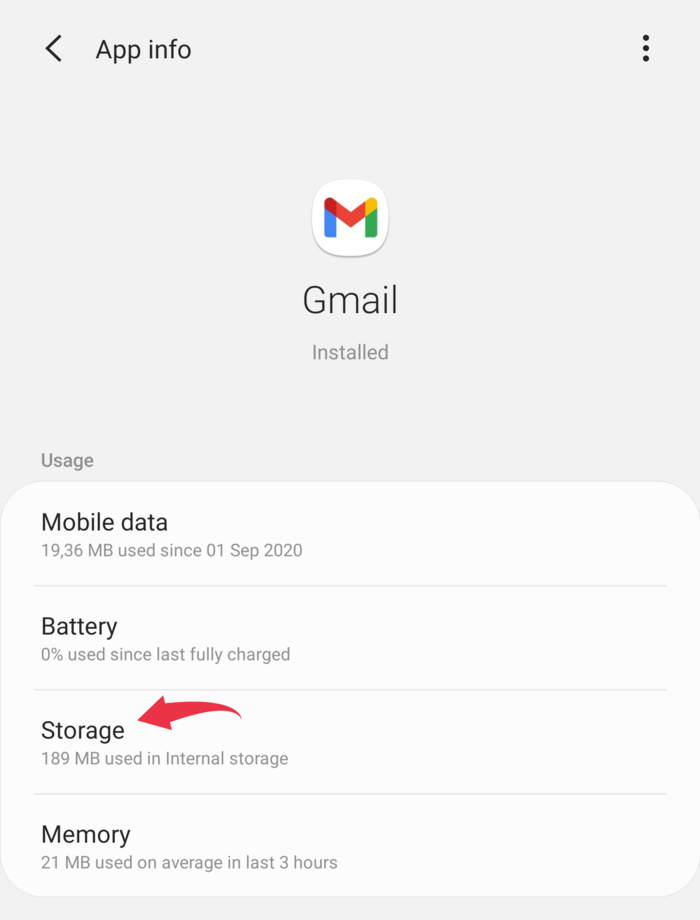**Web Pages**

The image depicts a detailed application information screen for the Gmail app. At the top of the screen, there is a large grey header featuring a back arrow labeled "App Info" next to it, enabling navigation to the previous page. On the right side of this grey header are three vertical dots, which, when clicked, open a menu for additional options.

Centered within the grey header is the iconic Gmail logo, stylized as an envelope with sections colored blue, green, yellow, and red. Beneath the logo, "Gmail" is clearly printed, followed by the word "Installed."

Below this header, various usage statistics are displayed. The first line, labeled "Usage," showcases that "Mobile data" usage is 19.36 megabytes since 1 September 2020. The next category indicates that the battery has used 0% since it was last fully charged.

A prominent red arrow highlights the "Storage" category, which shows that Gmail occupies 189 megabytes of internal storage. Following this, the "Memory" section informs that the app has used 21 megabytes on average over the last three hours.

Each category title—Usage, Battery, Storage, and Memory—is presented in black letters within white boxes, while the actual data values (like megabytes used) are rendered in grey text, maintaining a consistent visual format.